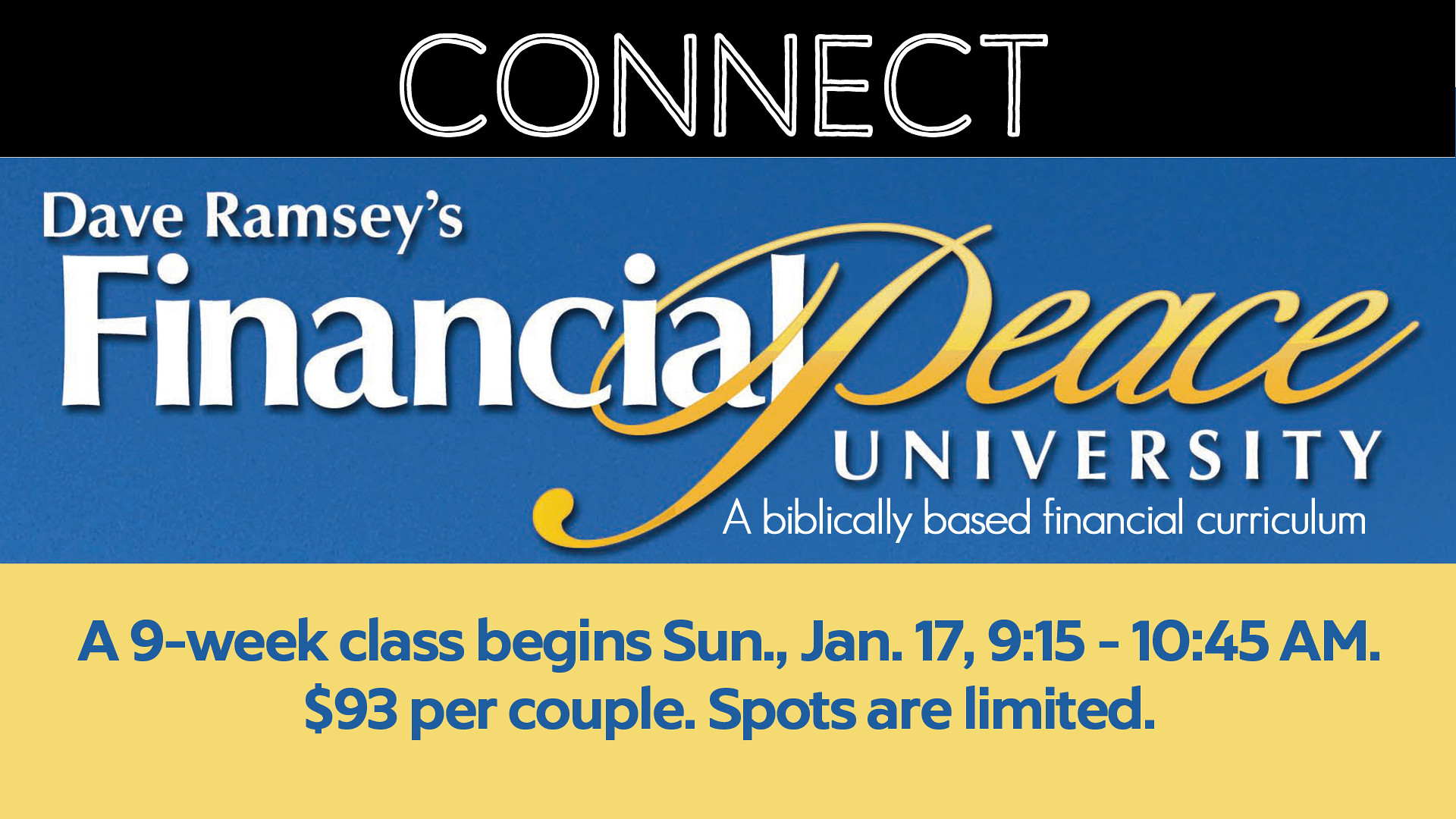The image is a promotional advertisement designed like a business card, divided into three distinct sections with different colors. At the top, there is a narrow black strip featuring the word "CONNECT" in bold, white, capital letters centered in the middle. The central section is a large blue strip showcasing the logo and text "DAVE RAMSEY'S FINANCIAL PEACE UNIVERSITY, a biblically based financial curriculum," written in white. The bottom section is a medium-sized yellow strip with blue text stating, "A nine-week class begins Sunday, January 17, 9:15 to 10:45 AM. $93 per couple, spots are limited," with the phrase "spots are limited" emphasized in cursive.